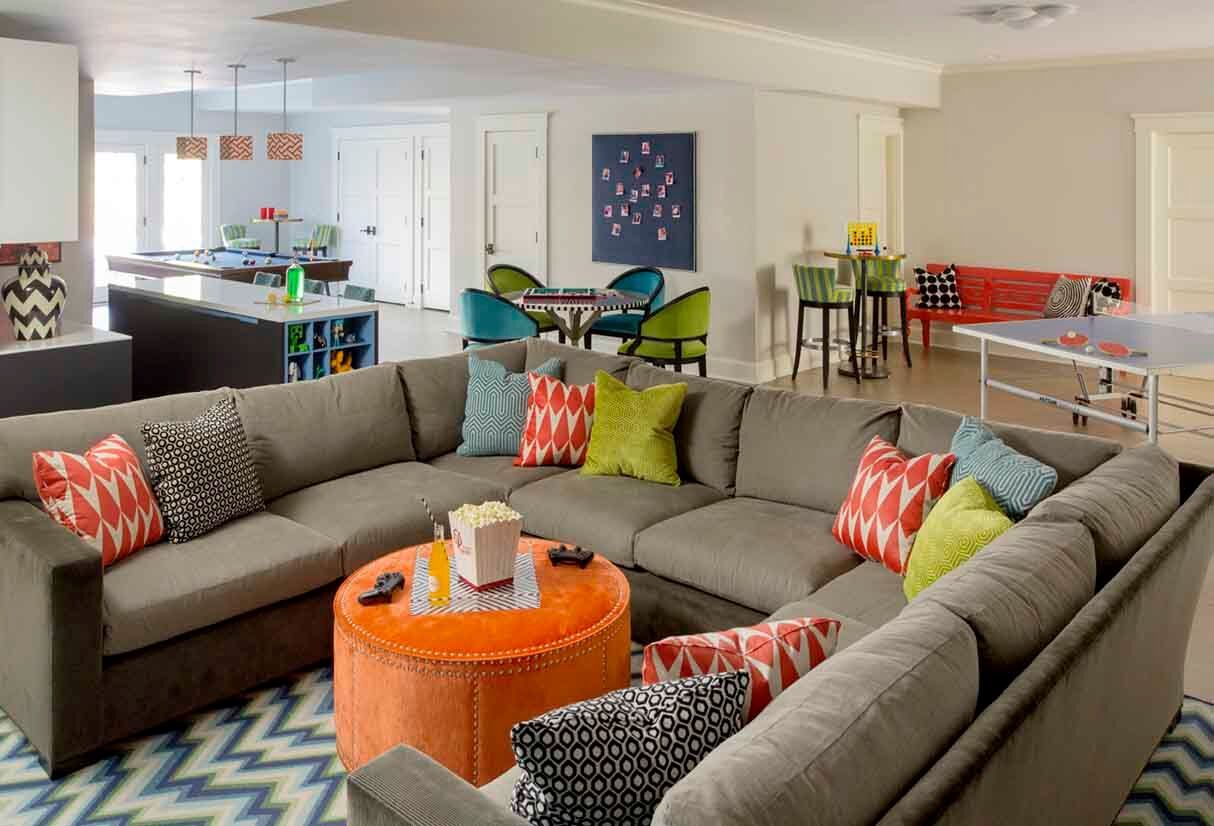This image depicts a vibrant and multifunctional living room designed for entertainment and relaxation. Dominating the center of the room is a large U-shaped gray sectional couch adorned with an array of multi-colored pillows featuring various patterns, including greens, dark blues, teals, lime greens, and some shades of orange, red, black, and white. These colors and patterns resonate throughout the room's décor. 

In front of the couch stands an eye-catching coffee table upholstered in orange, serving as a central hub with a bucket of popcorn and orange soda, alongside a pair of gaming controllers indicative of the room's recreational purpose. The coffee table is described alternately as both a leather-looking ottoman and a large, round, brown piece, adding to the eclectic mix of textures and styles.

The background is equally engaging, showcasing a ping-pong table, a pool table with scattered balls, and a variety of seating arrangements, including benches and loungy chairs around a round table, ideal for board games or casual gatherings. The room features additional playful elements like a red bench with black and white spots, a white and black vase, and colorful pops that enhance its lively ambiance.

Overhead, square lights provide illumination, while natural light streams in from doors located on both the top left and right sides of the room. The walls maintain a consistent gray tone, tying together the colorful and patterned elements seamlessly. This living space is clearly designed as a versatile and inviting area, perfect for entertaining guests and unwinding with activities.